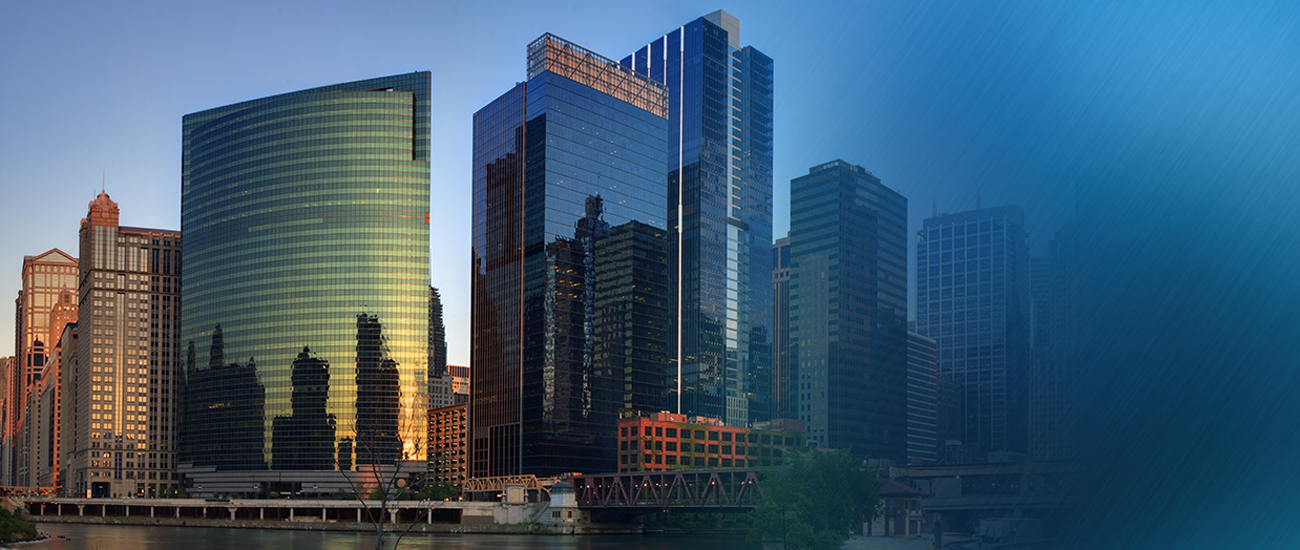This is a detailed photographic image of a city skyline taken during the early morning. The setting is outdoors under a clear blue sky with no visible clouds. The image is centered on a collection of tall skyscrapers, characterized by their glassy, reflective surfaces. The buildings are mostly glass and metal, with one prominent bronze-tinted glass building on the left that features a rectangular shape with a gabled roof. Adjacent to it is a tall, stone-structured skyscraper partly obscured by another multi-story glass building with a slightly inclined roof.

As your eyes move from left to right in the photo, the clarity of the scene diminishes. The right-hand section appears smoky, hazy, and is heavily faded, almost as if there was something on the camera lens. The very far right of the image turns into a solid, hazy blue, likely an effect of the photo rather than natural weather conditions. Among the array of buildings, there is also a smaller, older brick building about three or four stories high and another skyscraper with unreadable text on it.

At the ground level, in the foreground, you can see a body of water, likely a large river, bordered by what looks like a concrete roadway and an iron or metal bridge stretching across it. The reflections of other buildings can be seen in the glass surfaces of the skyscrapers, accentuating the clean lines and modern aesthetics of this urban panorama. The light reflecting off the buildings and the low shadows indicate that this photo was taken either early in the morning or late in the evening.